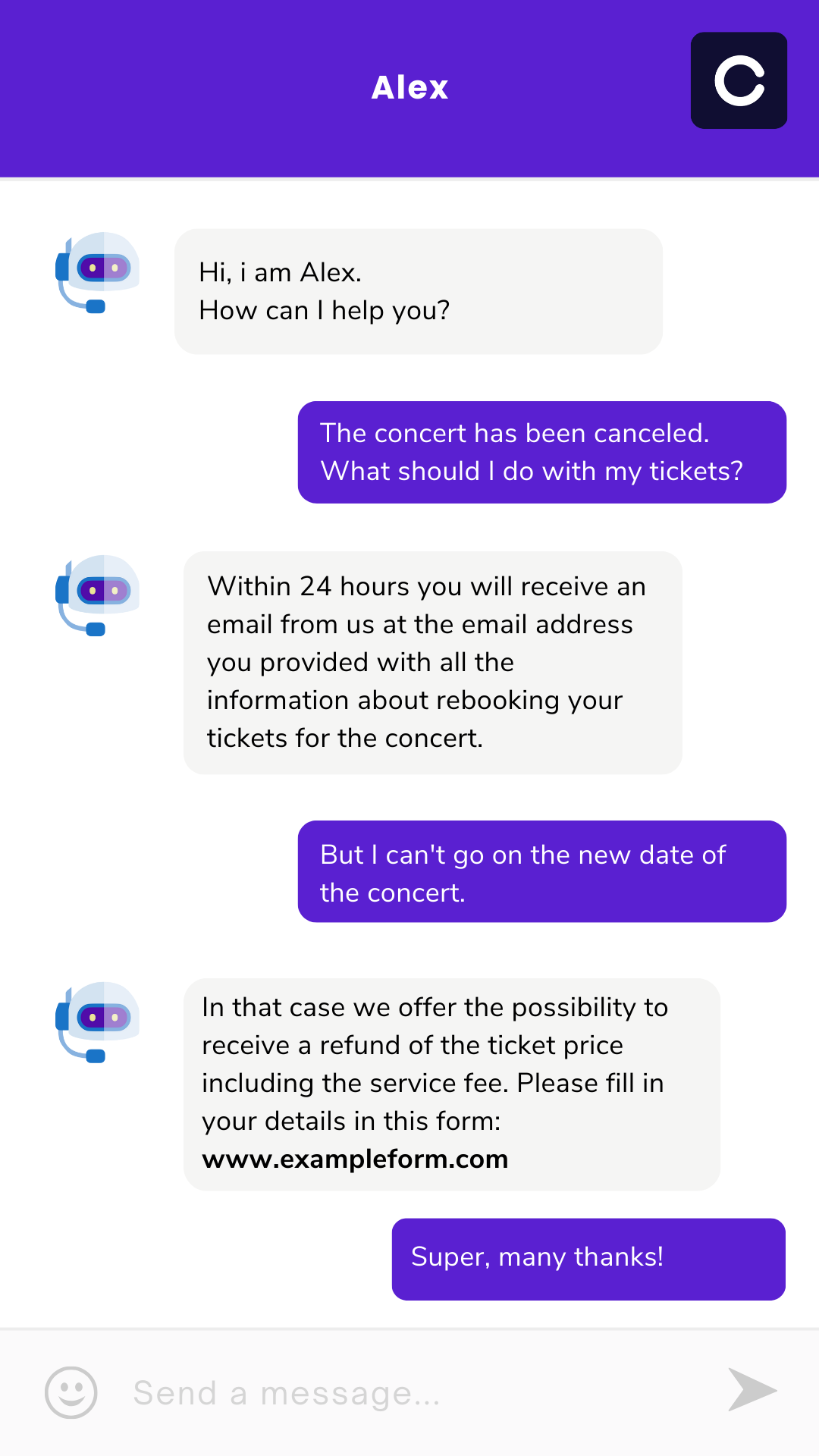In the top portion of the image, a rectangular purple banner is featured. Centered within this banner, the name "Alex" is prominently displayed in white text. Below this, there's a black square containing a letter "C" or a similar shape resembling part of a circle.

To the left, an image of a robot is present. Adjacent to this robot, a gray rectangle with rounded corners contains the text, "Hi, I'm Alex, how can I help you?"

Following this, there is another purple rectangle with rounded corners that states, "The concert has been cancelled, what should I do with my tickets?"

Adjacent to this, yet another image of a robot appears. Beside it, within a gray rectangle with rounded corners, it reads, "Within 24 hours you will receive an email from us at the email address you provided with all the information about rebooking your tickets for the concert."

Next, a third purple rectangle with rounded corners states, "But I can't go on the new date of the concert."

Continuing along, another robot image is displayed. Beside it, a gray rectangle with rounded corners reads, "In that case, we offer the possibility to receive a refund of the ticket price including the service fee. Please fill in your details in this form: www.exampleform.com."

Lastly, a final purple rectangle with rounded corners expresses, "Super, many thanks."

Below these interactions, a light gray line divides the content. Underneath this line, a light gray rectangular box appears. On the left side of this box, a happy face icon is visible next to the text, "Send a message." On the right side, there is an arrow pointing to the right, indicating a prompt to proceed or send the message.